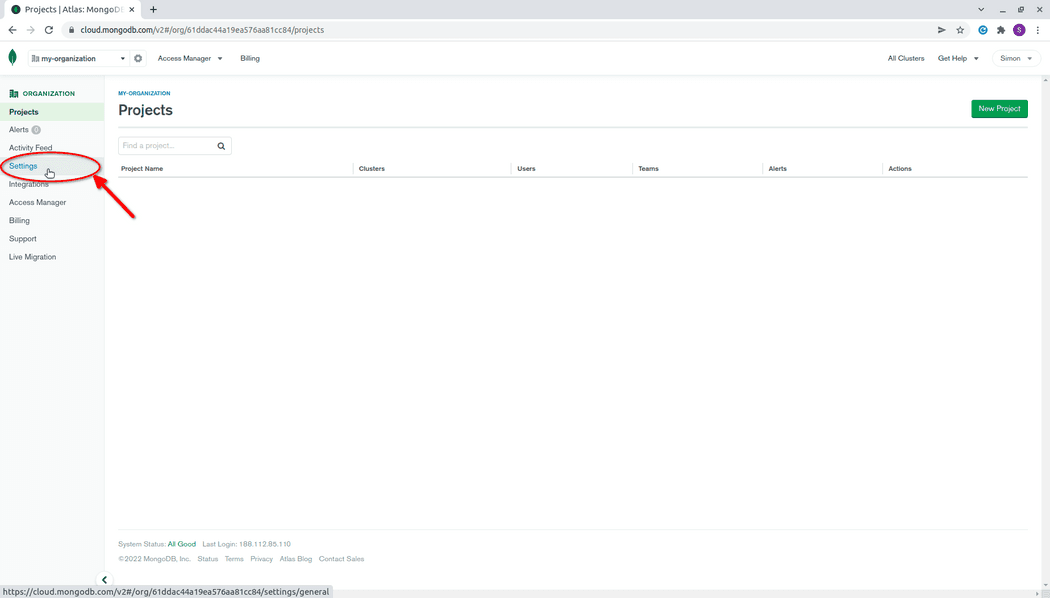The image depicts a screenshot of a website featuring a predominantly white background. At the very top of the browser tab, the word "projects" is displayed in black font, with the label "Atlas: Mongo" written in a faded style, indicating it is related to MongoDB.

On the left side of the webpage, there is a navigation pane. At the top of this pane, a green folder icon appears next to the word "organization," followed by the word "projects," which is highlighted in blue. Below that, unhighlighted, are the terms "alerts" and "activity feed." Further down, a list of options appears in small gray font: "integrations," "access manager," "billing," "support," and "live migration."

A blue-highlighted "settings" option is circled in red with a diagonal red arrow pointing towards it, and the mouse cursor, depicted as a hand icon, is situated inside this circle.

In the main body of the webpage, next to the navigation pane, the word "Projects" is presented in large black font. Next to this, there is a search box with a magnifying glass icon. The section below features six columns with headers: "Project Name," "Clusters," "Users," "Teams," "Alerts," and "Actions." These columns are separated by thin gray lines, but the body of the columns appears to be blank.

This thorough depiction captures the structure and layout of the website interface shown in the image.